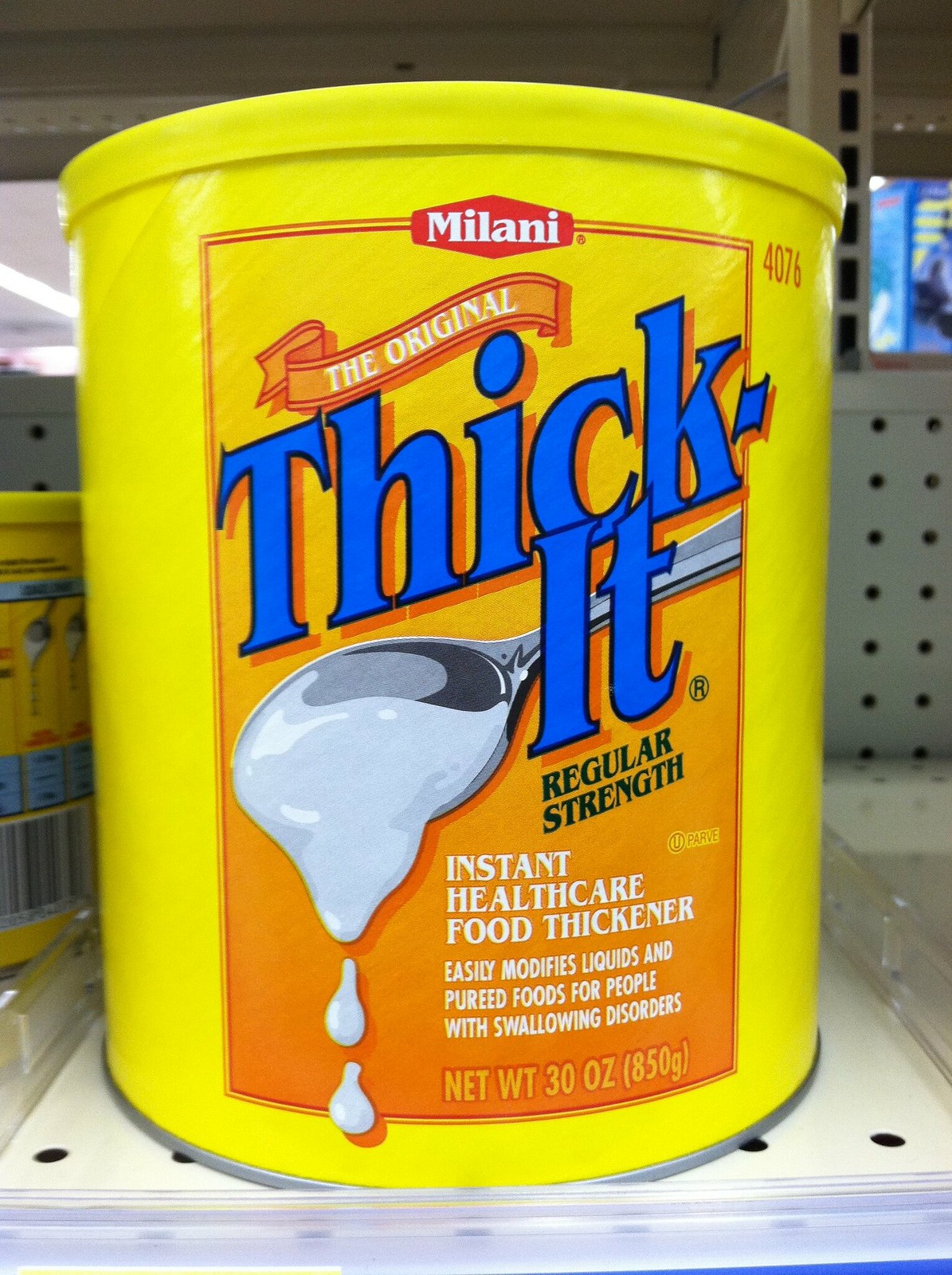This image features a round yellow container of "Thick-It" sitting on an off-white metal shelf, likely in a store or commercial facility, as indicated by the pegboard background. The container has a yellow lid, and prominently displays various labels and information.

At the top of the container, within a red box with white letters, it reads "Milani." Below that, an orange ribbon with white letters reads "The Original." The brand name "Thick-It" is displayed in large blue letters with an orange outline, accompanied by an image of a gray spoon dribbling white, thick liquid.

Underneath the brand name "Thick-It," in black letters, appears "Regular Strength." To the right of this, a registered trademark symbol (R in a circle) is visible. Further down, in white lettering, the container describes its contents as an "Instant Healthcare Food Thickener," which "easily modifies liquids and pureed foods for people with swallowing disorders."

At the bottom of the container, yellow letters indicate the net weight as "30 oz" (850 grams). Additionally, red numbers in the top right corner of the container indicate "4076," presumably a product or batch number.